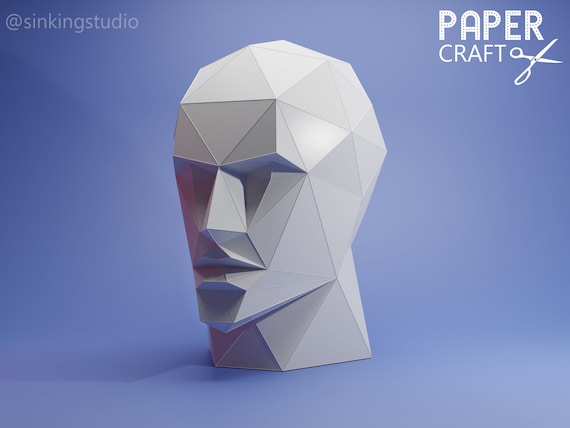The image features a highly detailed, computer-generated 3D rendering of a human head, composed entirely of interconnected gray triangles, giving it a distinctly geometric and angular appearance reminiscent of early 3D video game graphics or modern papercraft art. Set against a blue background, the face is distinctly three-dimensional, with the light source from the right side creating a lighter gray on the right and a darker shade on the left. Key facial features such as the eyes, nose, mouth, and pointy chin are clearly defined by the geometric pattern. In the top left corner of the image, the text "Sinking Studio" is displayed alongside an '@' symbol in white font, while the top right corner reads "PAPER CRAFT" in all capital letters with an illustration of open scissors, suggesting a connection to papercraft activities. The head is angled slightly towards the left, resting on a small block-like structure representing its neck.